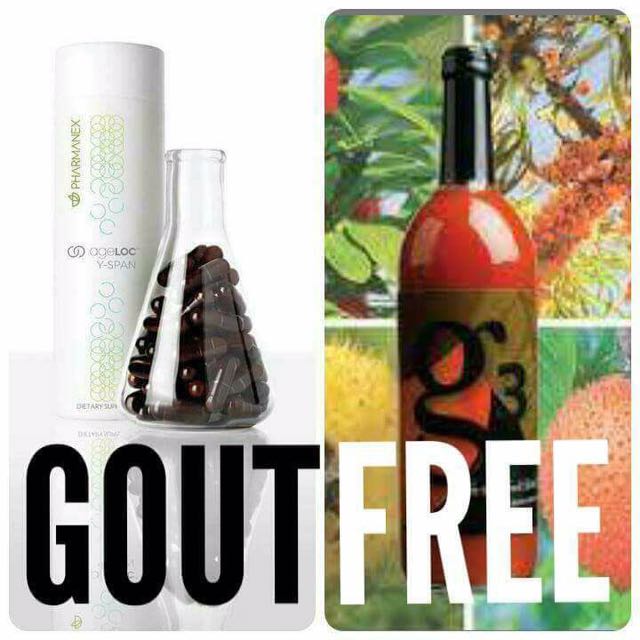The image is a low-resolution, two-panel advertisement with the overall theme "Gout Free." The left panel prominently features the word "GOUT" in bold black text at the bottom. This side displays a cylindrical white bottle with faint black lettering and a green logo that likely reads "Pharmanex." Next to the bottle is a scientific beaker filled nearly to the top with black or brown capsules, sitting on a stand. The right panel has "FREE" written in thick white text at the bottom. The centerpiece here is a bright red bottle with a greenish-red label that reads "G3" in black text, adorned with a black foil wrap commonly used for wine bottles. The background of the right panel is a patchwork of four different green and colorful quadrants: the upper left shows plants, the upper right is a mix of various colors, the bottom right features a close-up of a spiky reddish flower, and the bottom left displays a spiky yellow flower. Overall, the ad contrasts the two panels with their respective focal points and textual elements to convey a message of relief or solution.